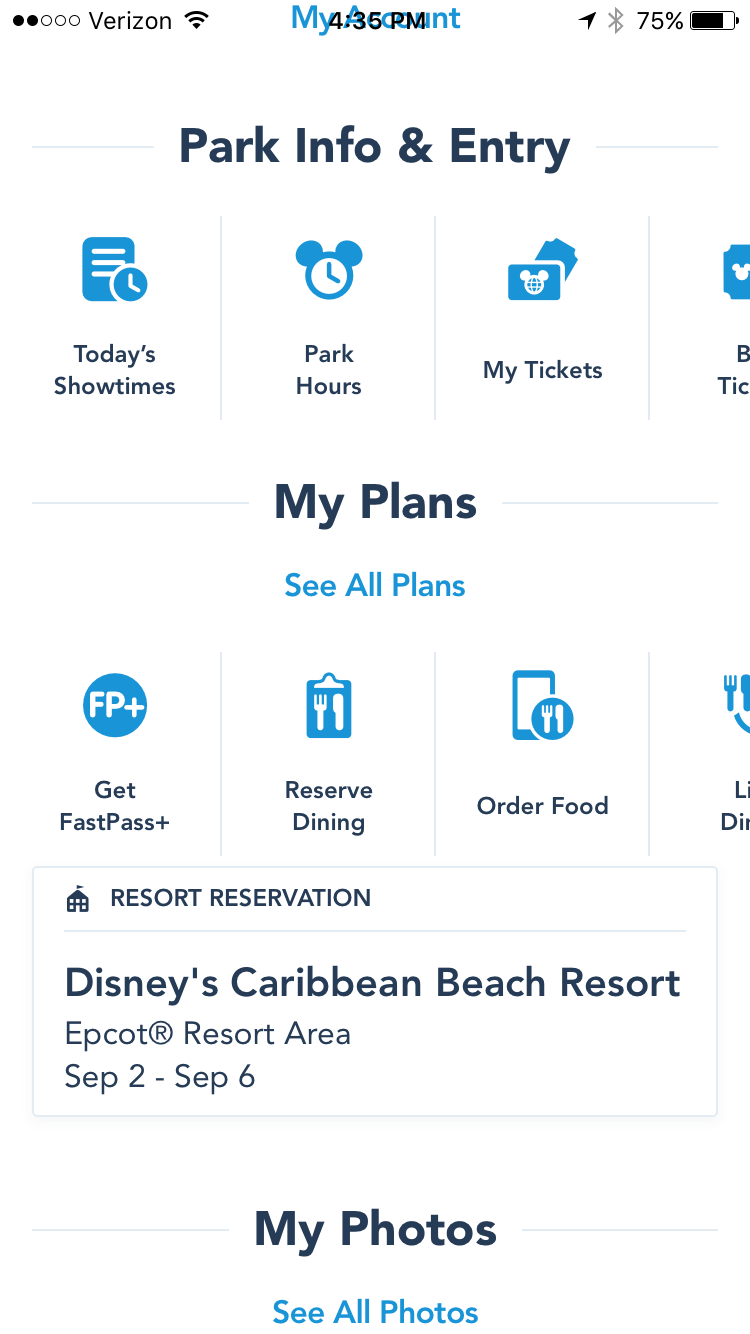This is a detailed mobile screenshot of a summary page for Disney's Caribbean Beach Resorts.

Across the top of the screenshot, two out of five circles are filled in black, indicating the cellular service strength provided by Verizon. Adjacent to this indicator is a fully filled Wi-Fi symbol with two bars. The time, 4:35, is displayed over the blue text "My Account," slightly obscuring the readability of both. To the right, various icons can be seen: a compass pointing to the northeast, a Bluetooth symbol, the text "75%" indicating battery percentage, and a battery icon reflecting a 75% charge in black on a white background.

The page theme is predominantly white, with black text and light blue icons. The first section, titled "Park Info and Entry," contains a row of four icons, although the fourth icon is partially cut off. The icons and their labels are as follows: 
1. "Today's Showtimes," represented by a piece of paper with three lines and a blue filled clock.
2. "Park Hours," shown as a clock with Mickey Mouse ears in blue.
3. "My Tickets," depicted as a wallet with a Mickey Mouse globe symbol and a ticket peeking out from the upper right corner.
4. A partially visible icon starting with the letter "B" and text below starting with "T-I-C," possibly indicating tickets or bookings.

Following this is the "My Plans" section with blue text "See All Plans" as a header. The icons here are:
1. "Get Fast Pass Plus," symbolized by white text "FP Plus" inside a blue circle.
2. "Reserve Dining," shown as a white fork and knife inside a blue clipboard.
3. "Order Food," depicted with a blue outline of a mobile phone with a white fork and knife inside a circle.
4. An icon cut off at the bottom, starting with letter "L" and the second word beginning with "D-I," possibly linked to dining, with a fork, knife, and maybe an arch underneath.

Below these sections is a divided box. The left side reads "RESORT RESERVATION" with a carnival tent icon, followed by the text "Disney's Caribbean Beach Resorts," "Epcot® Resort Area," and dates "SEP 2 - SEP 3." 

The final section, titled "My Photos," has the blue text "See All Photos."

This captures the organized layout and informational elements of the page, with a focus on icons and sections relevant to park info, personal plans, reservations, and photos.